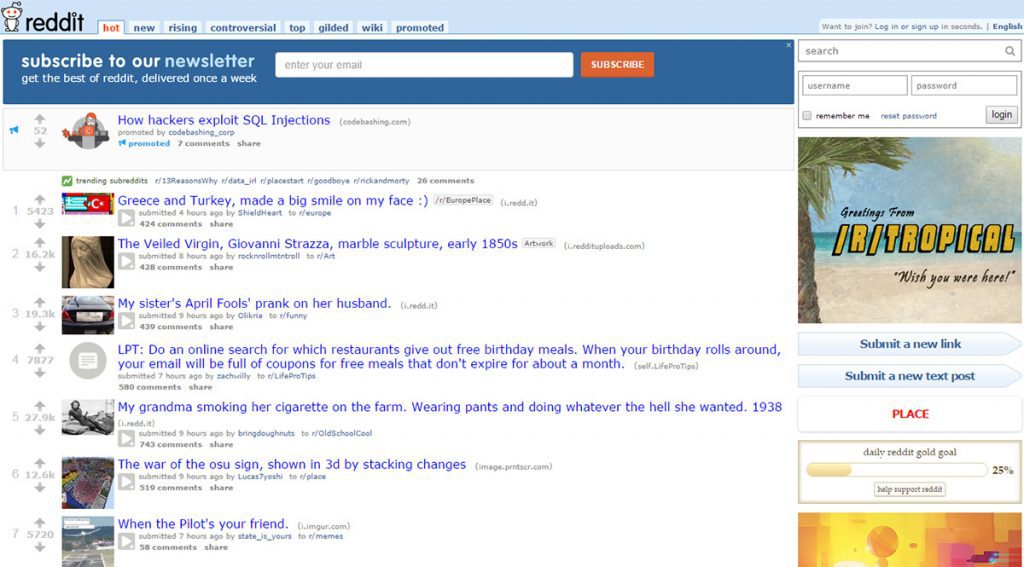In this image, we see a detailed screenshot from Reddit. In the upper left-hand corner, several tab options are visible, including "Hot," "New," "Rising," "Controversial," "Top," "Gilded," "Wiki," and "Promoted." Below these tabs, there is a banner inviting users to "Subscribe to our newsletter" to get the best of Reddit content delivered once a week. A text box for entering an email and a "Subscribe" button are also shown.

The post at the top of the feed is titled "How Hackers Exploit SQL Injections." Following that, the next post reads "Greece and Turkey Made a Big Smile on My Face." The subsequent post features "The Veiled Virgin" by Giovanni Strazza, a marble sculpture from the early 1850s. Down the list, another post highlights "My Sister's April Fool's Prank on Her Husband."

Further down, there is a Life Pro Tip (LPT) post suggesting, "Do an online search for which restaurants give out free birthday meals. When your birthday rolls around, your email will be full of coupons for free meals that don’t expire for about a month."

Next is an image post titled "My Grandma Smoking Her Cigarette on the Farm, Wearing Pants and Doing Whatever the Hell She Wanted, 1938." This is followed by "The War of OSU Sign Shown in 3D by Stacking Changes," and the final post at the bottom says, "When the Pilot's Your Friend."

The image encapsulates diverse Reddit content, ranging from educational posts and personal stories to historical photos and practical life tips.